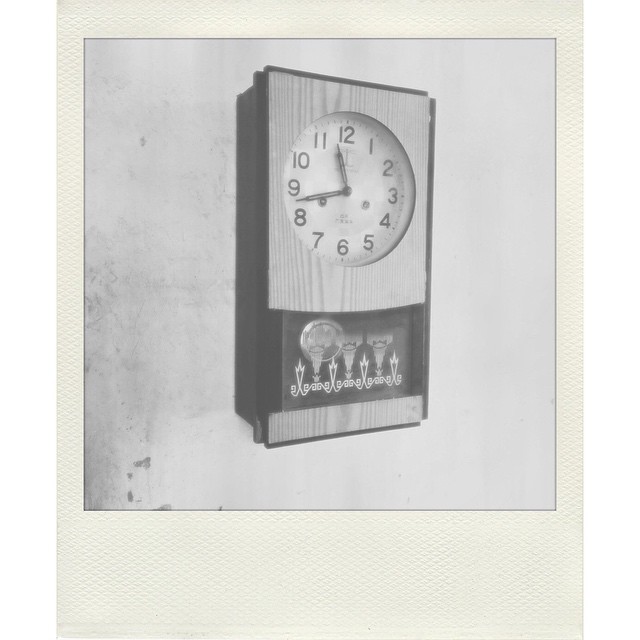A beautifully composed black-and-white photograph centers on an antique clock. The clock, with its rectangular wooden case, boasts a classic design, complete with a pendulum visible through a glass panel at the bottom. The clock face, set within the wooden frame, features large numerals from 1 to 12 and black-and-white hands that enhance its vintage appeal. The backdrop of the image is a plain white card with a distinctive checked texture, adding depth and context to the central subject. The juxtaposition of the textured card against the old-fashioned clock creates a compelling visual, capturing the essence of timeless elegance.